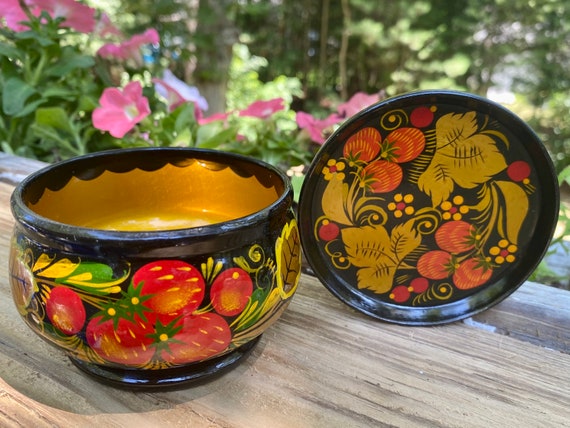This is a color photograph taken outdoors during the daytime, depicting a black acrylic bowl and its matching lid resting on a light brown, wood-grain picnic table. The bowl features hand-painted designs of red fruits, likely tomatoes, with green stems and leaves. The rim of the bowl is black, with its interior side painted a rich gold. Similarly, the lid, standing upright on the right side of the image, showcases a black background adorned with similar red fruit, green leaves, and gold filigree designs, including some gold teardrops and spiral elements. The backdrop reveals a natural setting with some bushes on the middle left that have pink flowers and larger trees with green leaves on the top and right sides of the image. The bowl appears slightly water-damaged, and no text is present in the image.